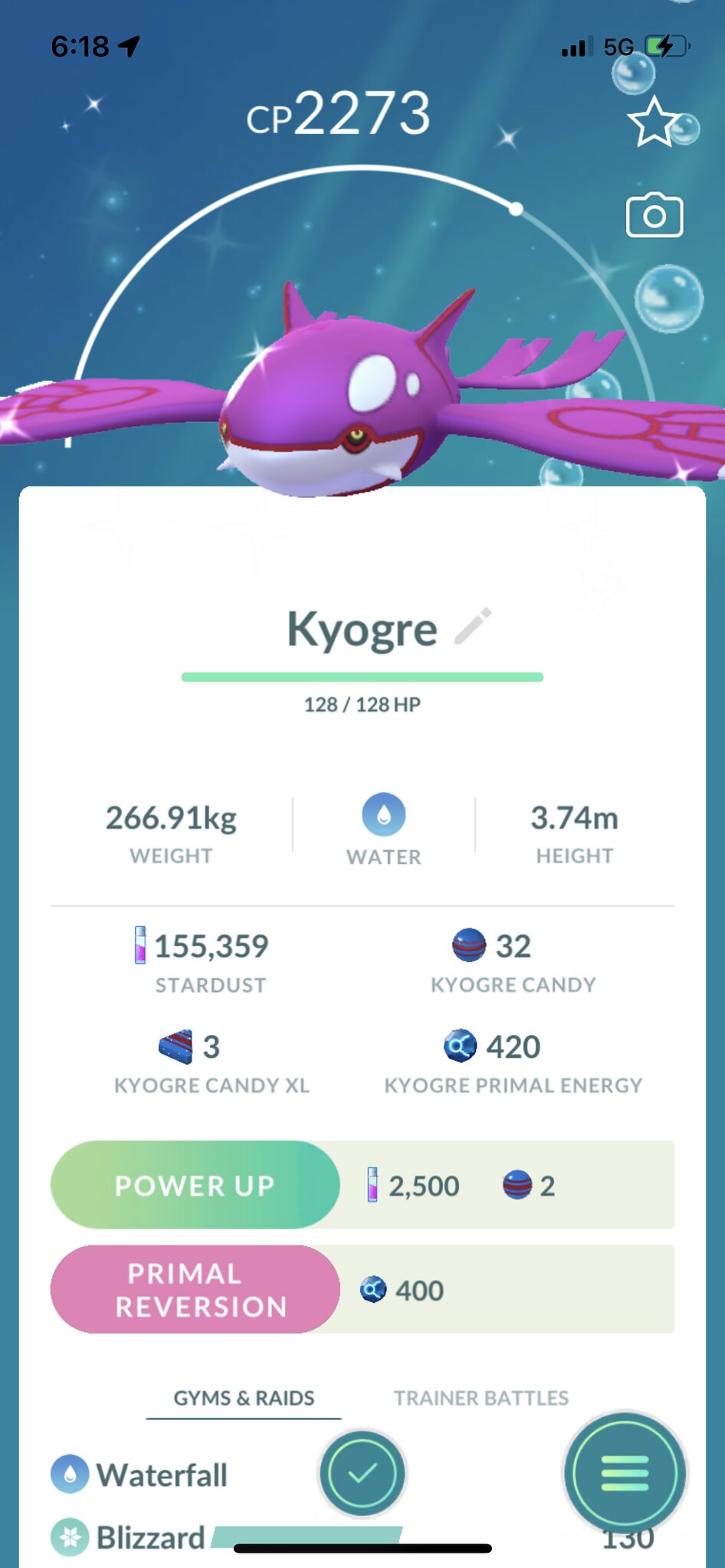This image is a vertically oriented screenshot from a smartphone displaying details of a Pokémon Go character named Kyogre. In the top left corner, the time reads 6:18, and the top right shows the phone's status indicators, including a 5G signal with three out of four bars and a partially filled green battery symbol. The background features a blue sky with stars and dots. Centered in the image is Kyogre, a Pokémon that resembles a pink whale with cat ears and wide, wing-like fins. The Pokémon has large white eyes and is identified at the top with the name "Kyogre" in black text. Beneath the name, a green line indicates its full health at 128/128 HP. Further details include Kyogre's weight of 266.91 kilograms, a water symbol signifying its type, and a height of 3.74 meters. Other statistics shown are the amounts of Stardust, Kyogre Candy, Kyogre Candy XL, and Kyogre Primal Energy. There are buttons labeled "Power Up" and "Primal Reversion," with options at the bottom for "Gyms & Raids" on the left and "Trainer Battles" on the right.